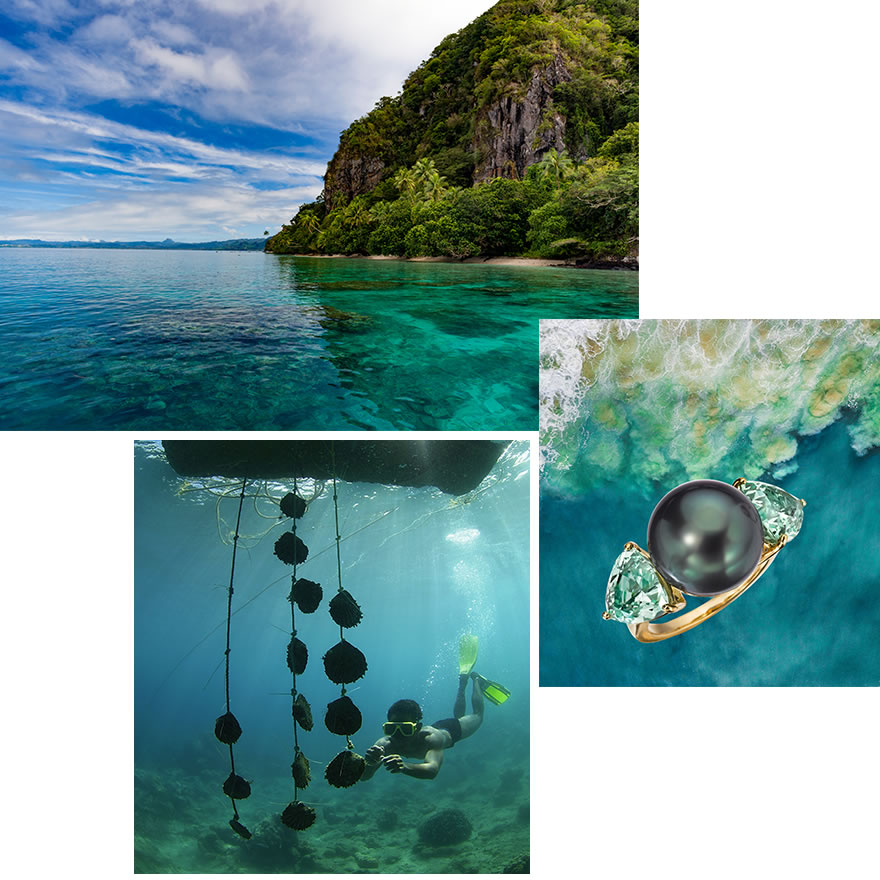This collage of three photographs provides a vivid view of a picturesque coastal scene. The largest image at the top captures a stunning lagoon or bay, likely in an isolated island region such as the South Pacific or near Thailand. The landscape features a beautiful beach edged by cliffs and lush green foliage with coconut trees. A mountain rises to the right, set against a brilliant deep blue sky adorned with fluffy clouds. The horizon reveals more of the land, gently sloping and majestically distant, while the water below is a pristine, clear blue that invites a sense of serene depth.

Below this, to the left, is a captivating underwater scene of a boy in a yellow mask, black swimming pants, and green flippers. He dives towards lines of shellfish – possibly clams or oysters – strung up below the water’s surface, in what appears to be the murky blue and green depths near the bottom of a boat. The natural sunlight penetrates the water, revealing green rocks and a rugged seabed.

To the right of the underwater image is a close-up photograph of an exquisite black pearl ring. The central black pearl is set in a gold band, flanked by two aquamarines in a triangular shape on each side. This elegant piece of jewelry is juxtaposed against a background of the same clear turquoise waters, highlighted with touches of white from the sunlight reflecting off the waves. Together, these images weave a detailed and immersive narrative of natural beauty and underwater exploration.